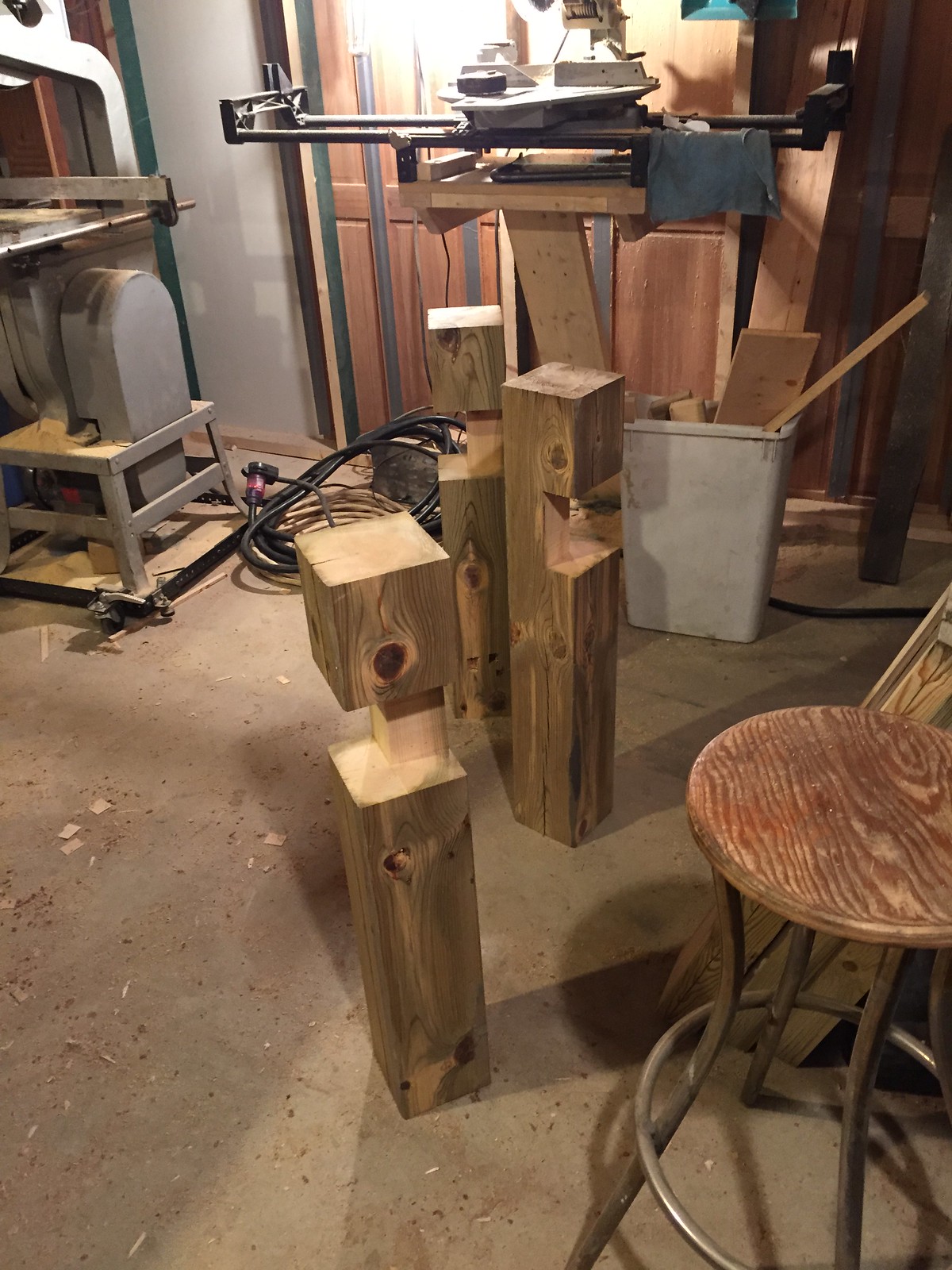The image depicts a workshop-like indoor space, possibly a garage or a basement, with woodworking activities evident throughout. In the background, a wooden door with a window stands, illuminated by a light source shining above it. A prominent silver table saw, used for cutting wood, sits to the left side of the background. Below the saw, a collection of thick black electrical cords snakes across the floor. Dominating the right foreground is a stool with a well-worn wooden seat and steel legs.

Centered among the scattered woodpieces is a white plastic trash can filled with variously sized cut boards. Nearby, three accurately cut pieces of lumber, each about two feet tall, exhibit intricate 90-degree cut-outs reminiscent of Lincoln Logs, indicative of assembly work requiring precise cuts. Additional wood of similar dimensions leans against the right-hand side, and the entire floor is peppered with wood chips and sawdust, hinting at ongoing or recent woodworking projects.